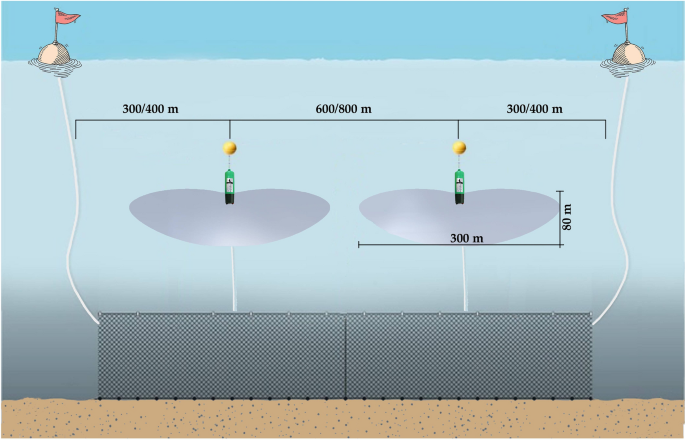This detailed CG diagram illustrates an underwater diving setup, showcasing various components and measurements. At the top, two buoys, each adorned with red flags, float on the water's surface, positioned at the extreme left and right sides of the image. From these buoys, white cords descend into the water, extending down to the ocean floor, where they attach to black rectangular tanks. These cords, measuring 300-400 meters long, anchor the tanks in place.

Further details emerge beneath the water's surface, revealing the ocean's blue gradient transitioning into a sandy brown seabed. Connected to the tanks are two white air bladders, each prominently displayed in the center of the diagram. Attached to these bladders are green canisters, each fitted with an orange balloon and situated directly below a yellow circle.

The diagram includes various measurements: the distance between the air bladders is 600-800 meters, while the individual bladders measure 300 meters wide and 80 meters tall. Additionally, there is a white-gray cloud emanating from the canisters, although its specific function is unclear. Overall, the image offers a comprehensive view of the underwater apparatus, highlighting the spatial relationships and dimensions critical to its design.